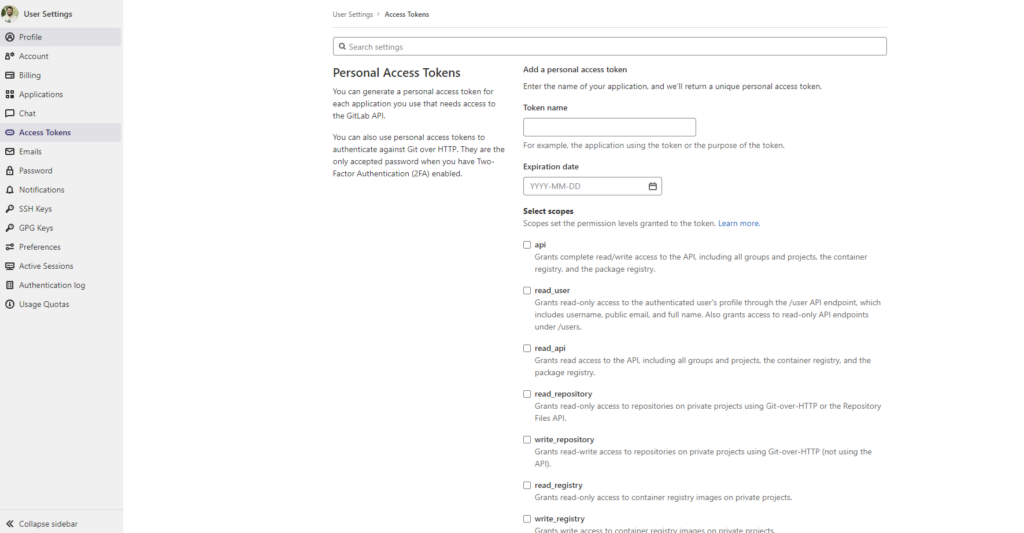A detailed screenshot of a website's backend interface, showcasing the user settings section. The layout features a gray sidebar on the left and a white main content area on the right. The gray sidebar includes a circular profile picture at the top, followed by the label "User Settings." Each navigation option on the sidebar is paired with a corresponding icon to its left and includes labels such as Profile, Account, Billing, Applications, Chat, Access Tokens, Emails, Password, Notifications, SSH Keys, GPG Keys, Preferences, Active Sessions, Authentication Log, and Usage Quotas.

In the main content area, the top section features two buttons labeled "User Settings" and "Access Tokens," with a breadcrumb navigation trail beneath them. Below this, a white search bar is prominently displayed, followed by a section titled "Personal Access Tokens" with a textual description providing additional information. The entire layout is clean and organized, aimed at facilitating easy navigation and management of user settings.